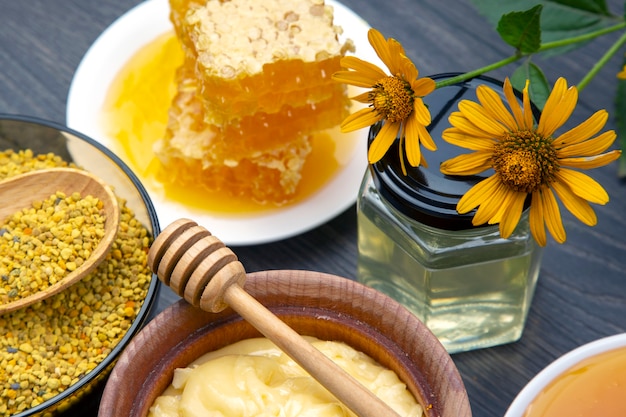In this vibrant photograph of a healthy breakfast setup, various items are meticulously arranged on a dark, grayish wooden panel table, enhancing the natural aesthetics of the scene. 

Starting from the far left, there's a clear glass bowl filled with bee pollen, described as tiny yellow granules with occasional green and orange specks. A large wooden tablespoon rests in the bowl, scooping up some of the pollen. Directly above this bowl to its right, a white plate showcases three sections of golden-orange honeycomb, glistening with dripping honey which pools at the base.

Moving further to the right, a clear hexagon-shaped jar with a black lid contains water, and inside it, two daisies add a touch of color and decoration. Below this, in the central lower part of the photograph, a wooden bowl holds what appears to be golden melted butter. Atop this bowl lies a wooden honey dipper, typically used for drizzling honey, suggesting the ingredients are being prepped for a honey butter spread.

In the lower right corner, the edge of a white plate is visible, partially filled with golden honey, adding to the overall appeal of the fresh and appetizing setup.